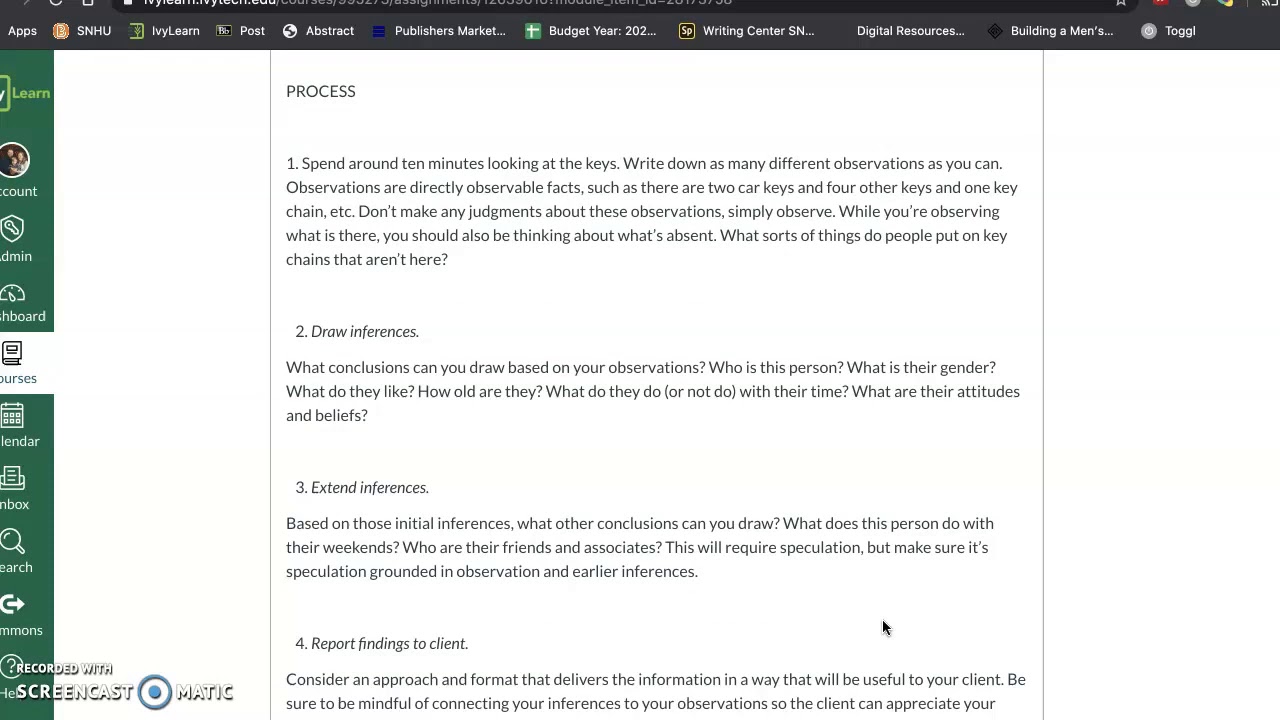The image depicts a digital interface, likely a web application, with a distinct black border at the top signifying a browser window. The browser's bookmark bar is present but appears small and blurry, becoming less legible when zoomed in. On the left side, a vertical sidebar lists several options, including Search, Inbox, Calendar, Dashboard, Admin, and Account. To the right of this sidebar, a prominent white box draws attention with the heading "Process."

The contents of the white box provide a detailed activity prompt:
1. Spend around 10 minutes examining the keys attentively.
2. Document numerous observations about the keys, focusing strictly on observable facts, such as noting the presence of two car keys, four additional keys, and a keychain.
3. Avoid making judgments or assumptions about these observations, focusing solely on the tangible elements.
4. Additionally, consider what is missing from the keychain, pondering items typically found on keychains that are not present, to form further inferences.
5. Conclude observations by speculating about the key owner: their identity, gender, characteristics, age, and lifestyle based on the gathered information.

This descriptive breakdown offers insight into the web application’s layout and the detailed instructions contained within, encouraging thorough analysis and critical thinking about an individual based on simple, everyday objects.